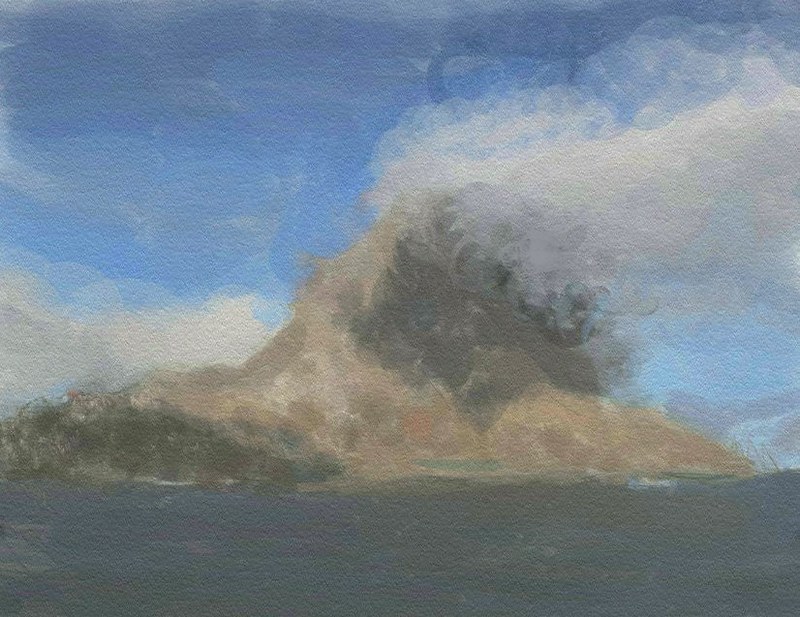A majestic, brown mountain rises prominently in the foreground, with its rugged slopes bathed in earthy tones. Shrouded in wisps of smoke that seem to curl around its peak, the mountain exudes an aura of mystique. The sky above is a gradient of deep blue at the zenith, transitioning to lighter blue and white hues as it descends. To the left, fluffy clouds drift lazily, adding a serene touch to the scene. The mountain's summit is capped with a dusting of white, possibly snow, contrasting sharply with the subdued gray ground below. Billowing clouds encircle the top, adding to the dramatic and almost ethereal atmosphere of the landscape.